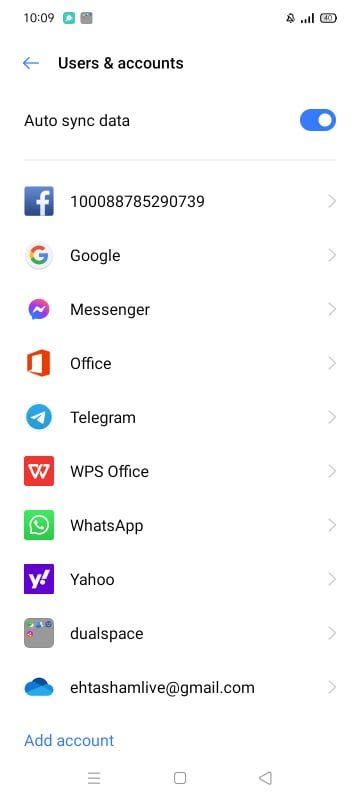**Detailed Image Description for Accessibility:**

The image depicts the "Users and Accounts" settings screen on a mobile device. At the top, the status bar shows the time "10:09" along with several icons. On the left, there's a small green square with a white dot inside it. Next to it is a gray square containing red and blue dots. To the right, there is a black bell icon with a line through it, signaling notifications are silenced. Following this, there are black signal bars indicating cellular reception strength and an outline of a battery showing "40%". 

Below the status bar, the header reads "Users and accounts" in black font with a blue arrow pointing to the left, leading back to the previous screen. Beneath this, the "Auto-sync data" toggle switch is prominently displayed; it is blue and white, indicating it is turned on.

A thin gray line divides this section from the list of accounts linked to the device:

1. **Facebook:** The emblem is a blue square with a white "F". The account ID displayed is "100088785290739" in black text, with a small gray arrow pointing to the right.
2. **Google:** Represented by a white circle containing a multicolored "G". 
3. **Messenger:** Shown by a chat icon in blue and purple with a white zigzag line.
4. **Office:** Depicted by a red box with a white center. 
5. **Telegram:** Represented by a blue circle with a white paper airplane icon.
6. **WPS Office:** Shown as a red square with white downward-pointing triangles.
7. **WhatsApp:** Displayed as a green square with a white chat bubble and telephone icon.
8. **Yahoo:** Represented by a purple square with a white "Y!".
9. **Dual Space:** Depicted by a gray square with multicolored dots in red, green, blue, and black, resembling small tools.

At the bottom of the list, an email account is shown: **E-H-T-A-S-H-A-M live at gmail.com**, represented by three shades of blue clouds with a blue triangle next to it. Below it, the text "Add account" is highlighted in blue.

Finally, three horizontal gray bars, a small gray square, and a left-pointing gray triangle are visible at the bottom of the screen, likely representing menu options or navigation buttons.